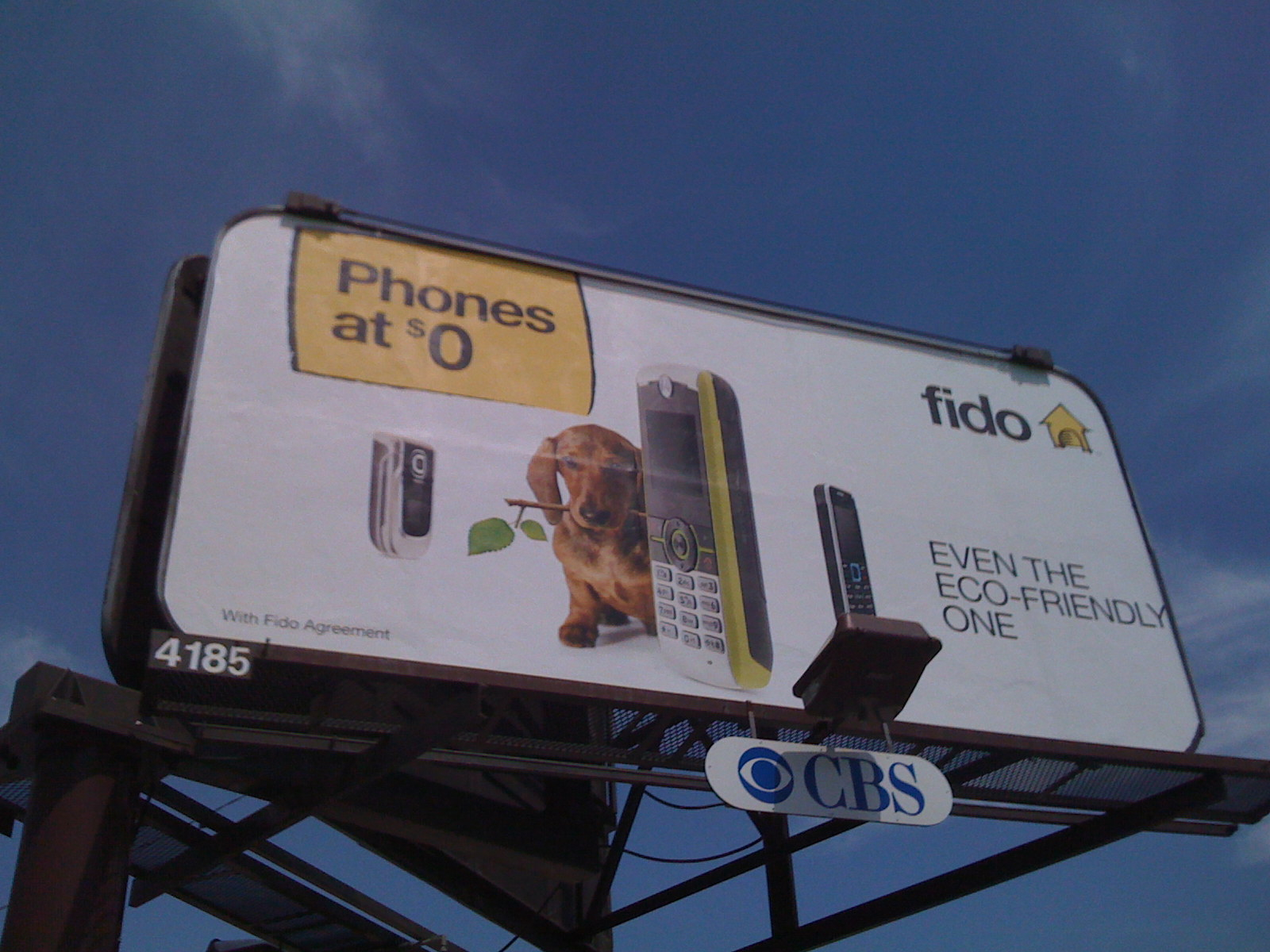This photograph captures a billboard advertisement for Fido, the phone carrier, viewed from the ground level against a backdrop of blue skies with light clouds. Dominating the center of the billboard is a yellow square that boasts "Phones at $0" in bold text. Below this headline, there is an image of a dog—specifically a sausage dog or dachshund—holding a twig with two leaves in its mouth. 

Next to the dog, centrally placed, is an old, brick-like mobile phone with a number pad, buttons, and a small screen. Flanking this phone, on the left, there is a flip phone, and on the right, a black candy bar-style phone. Positioned in the upper right corner, the Fido logo is featured with the word "Fido" and an accompanying doghouse icon. Near the bottom right, the text "even the eco-friendly one" is visible. 

At the lower edge of the billboard, there is another smaller sign displaying the CBS logo, which is blue on a white capsule-shaped background. This billboard is numbered 4185, as indicated in the bottom left corner. The structure supporting the billboard, including a graded platform used by workers, is visible at the bottom of the image, with a hint of another billboard seen from the back in the background.